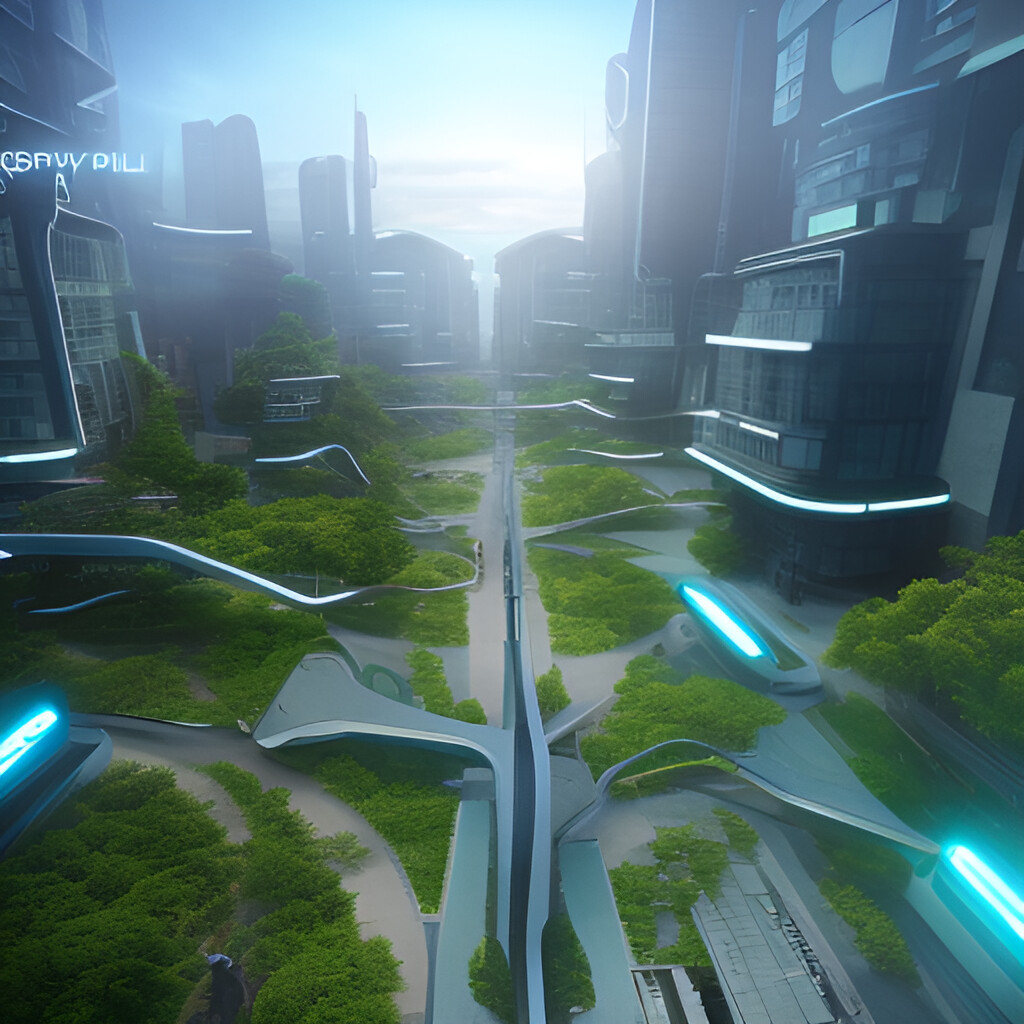The image depicts a digital rendering of a futuristic urban setting as seen from an elevated perspective. The scene features an intricate network of curving highways and ramps, glowing with bright turquoise neon lights, which contrast sharply with the typical flat roads of contemporary cities. Tall buildings, possibly residential skyscrapers, dominate the skyline, with some structures reaching impressive heights. In between these meandering highways, dense clusters of trees and shrubs add greenery to the landscape. The entire image is shrouded in a hazy atmosphere, muting the blue sky and lending a surreal, almost dreamlike quality to the futuristic cityscape.